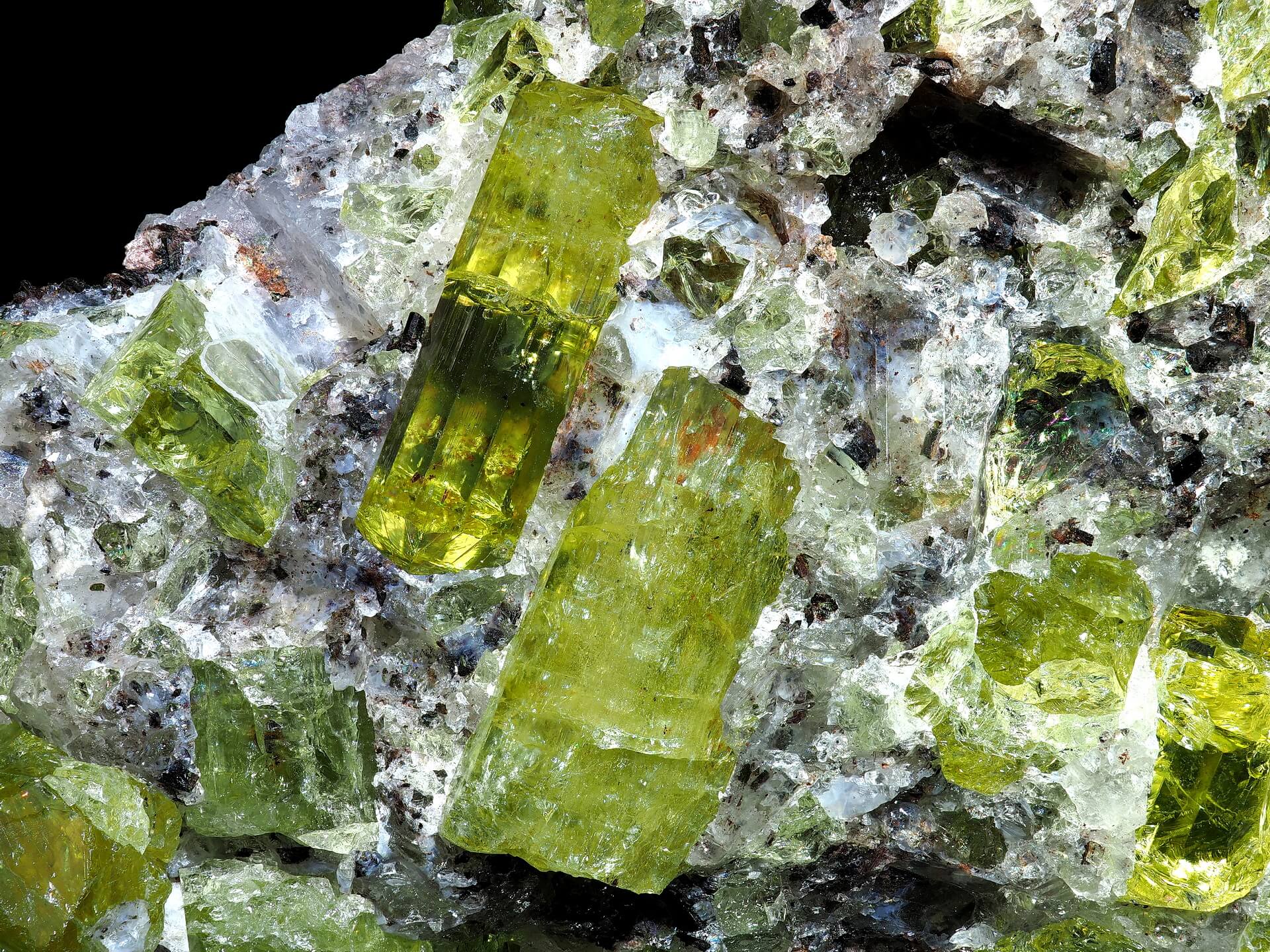This is a detailed, up-close photograph showcasing a cluster of 8 to 9 large green gemstones embedded in their natural matrix. The gemstones, which appear to be apatite crystals, are predominantly cylindrical in shape, resembling long pillars. They display a beautiful, translucent green color, reminiscent of chartreuse, with a crystalline texture similar to crushed ice. These distinctive crystals stand out against the surrounding rock, which features a combination of white, grey, and black hues with a somewhat shiny surface. The background of the photograph is completely black, enhancing the vibrant green and adding depth to the image. The composition highlights the beauty and natural arrangement of the gemstones within the matrix, creating a striking contrast between the crystals and their rough, speckled rock encasement.